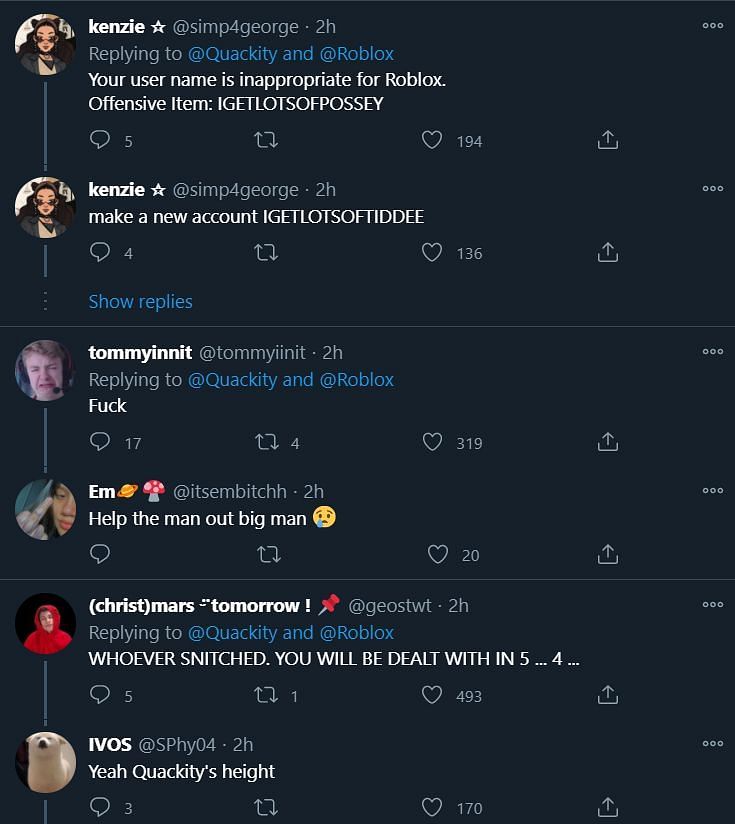In this image, we see a screenshot captured from a social media conversation, set against a black background. In the upper left corner, there is a profile picture of an anime-style character featuring a woman with black hair and pointy black ears. Next to this image, the username "Kenzie" is displayed in white text with a white star symbol following it. Directly below, the caption reads "@simpforGeorge, 2 hours ago" indicating the time of the post. The user is replying to "@quackity" and "@roblox", both mentioned in blue text.

Following this, the content of Kenzie’s message reads: "Your username is inappropriate for Roblox. Offensive item: I get lots of posse." This statement is just above five response messages.

Kenzie adds another message: "Make a new account, I get lots soft titty," which subsequently receives four replies.

Further down the thread, another user named "TommyInnit" replies to Quackity and Roblox with a succinct: "Fuck." TommyInnit's profile picture shows a photo of a man with brown hair.